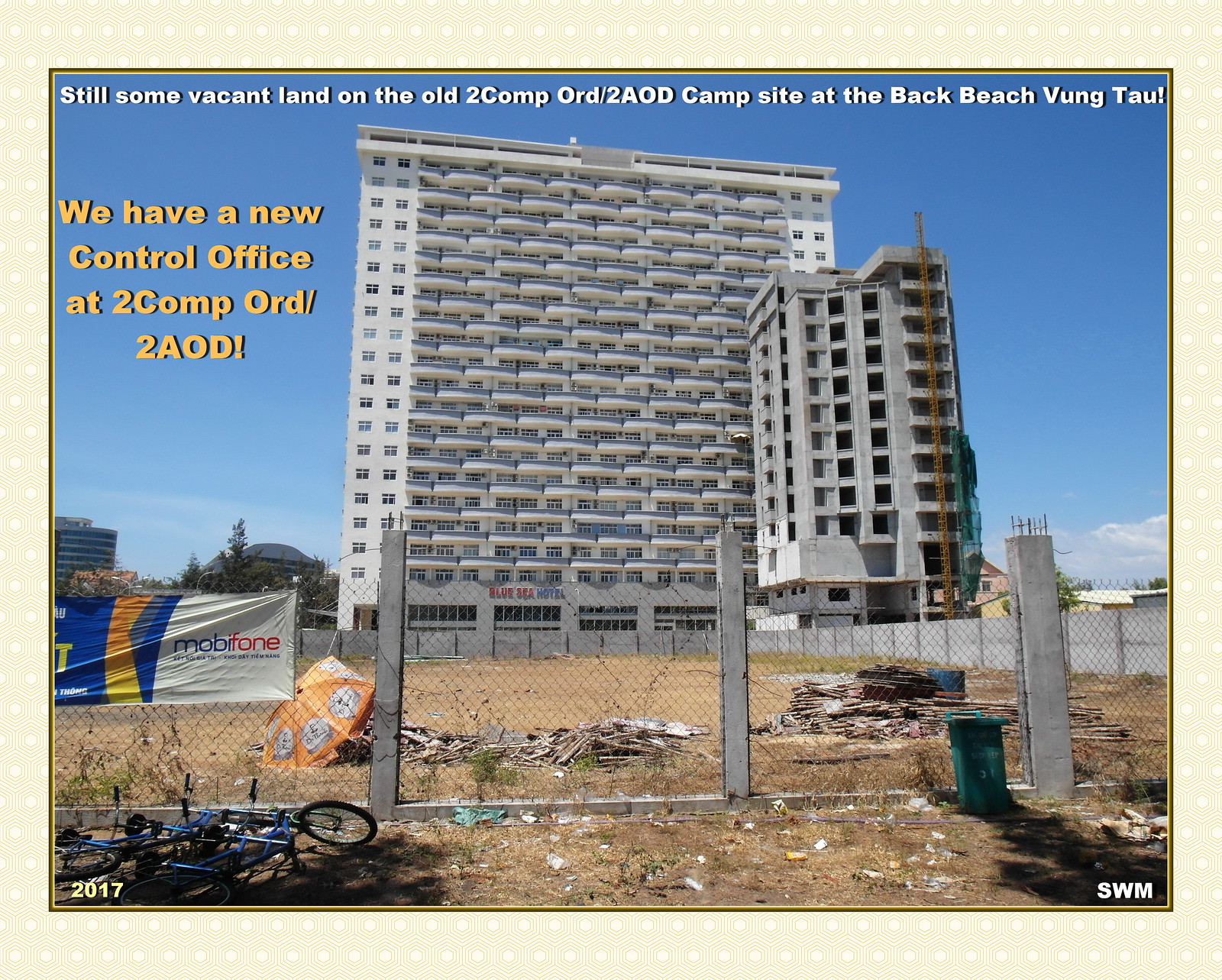This photograph captures a detailed view of a tall, multi-story building painted in white with numerous windows and balconies. Adjacent to it, a smaller, gray building under construction can be seen. In front of these structures lies an empty plot of land enclosed by a metallic chain-link fence. The ground within the fence is littered with debris, including old boards and construction materials, and dried brown grass covers the area. Concrete columns with exposed metal rebar stand among the debris, indicative of incomplete construction work. On the left side of the fenced area, several blue bicycles lie on the ground. Above, the sky is a vibrant blue, with white text reading "Still some vacant land on the old Tukomp/ORD slash 2AOD campsite at the Back Beach, Vung Tau." Additionally, in yellow text on the left, it says, "We have a new control office at Tukomp/ORD slash 2AOD!" Notably, the photo includes the year "2017" in the bottom left corner and the initials "SWM" in the bottom right corner.